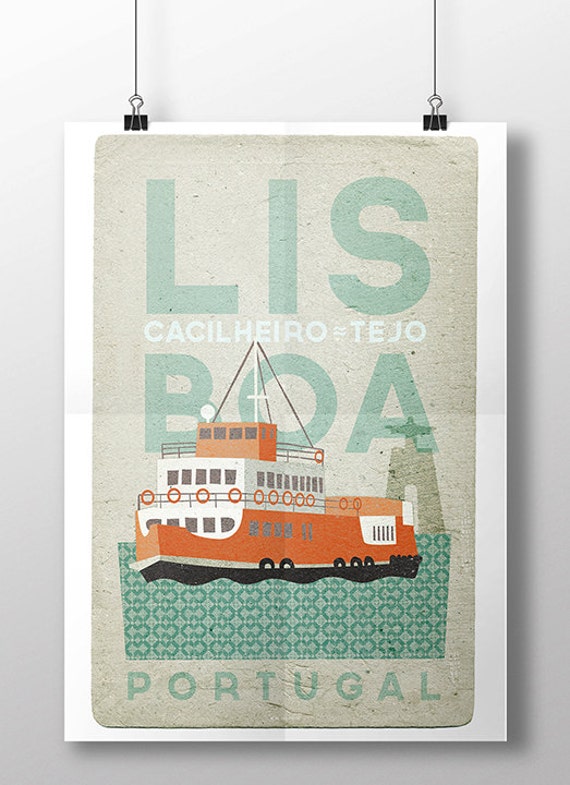The image depicts a poster hanging against a white wall, casting a subtle shadow. The poster is affixed by two black and silver clips with strings, visible at the top. Framed with a white border, the poster features a grayish-white background. Dominating the top section in large, pale green capital letters, it reads "LISBOA". Beneath this, in smaller white letters, the text "C-A-C-I-L-H-E-I-R-O T-E-J-O" is visible. Below the text is an illustration of a three-level boat, colored in orange and white, with black at the base and green, oval-shaped representations of water below it. The boat seems minimalist and cartoonish, with some lines extending from its top. At the very bottom, in pale green letters, the word "PORTUGAL" is prominently displayed.